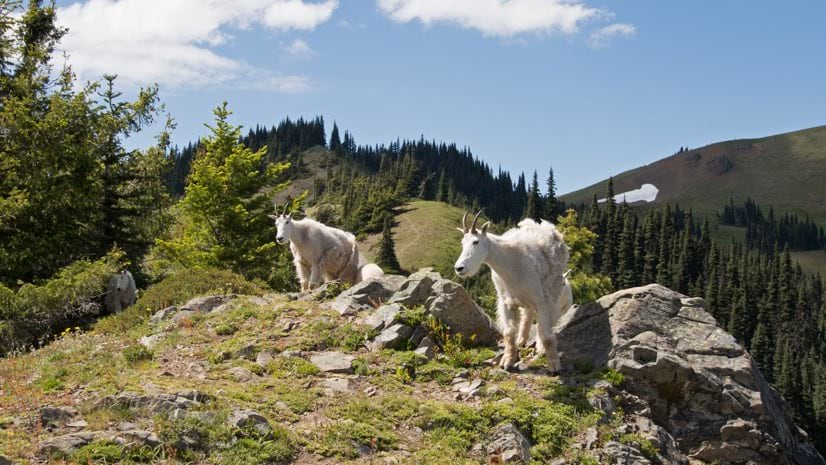This nature photograph features a detailed landscape with three prominent white mountain goats in the foreground, although only two are easily visible while the third is partially hidden behind some bushes on the left. These goats, with their distinctive shaggy fur and curved horns, are standing on rocky outcrops covered with patches of grass. One goat is slightly chunkier and positioned further back than the other.

In the midground, the landscape slopes downward revealing a line of tall, slender evergreen trees—likely some type of fir or pine—dotting the hillside. The foliage appears well-grazed, and faint paths through the grass hint at the goats' frequent activity in the area. The scene suggests a northern, possibly tundra climate, given the narrow shape of the trees and a slight hint of remaining snow in shaded areas.

The background extends into a series of hills and foothills, covered densely with green pine trees, further emphasizing the lushness of the area. A particularly striking large hill with exposed rocky formations rises towards the right, where the tree line recedes and occasional patches of snow are visible.

The sky above is a clear blue with scattered light clouds, indicating that the photograph was taken during the daytime. The composition of the image beautifully captures the rugged serenity of the goats' natural habitat, showcasing varied terrain, rich vegetation, and majestic evergreen trees across different elevations.